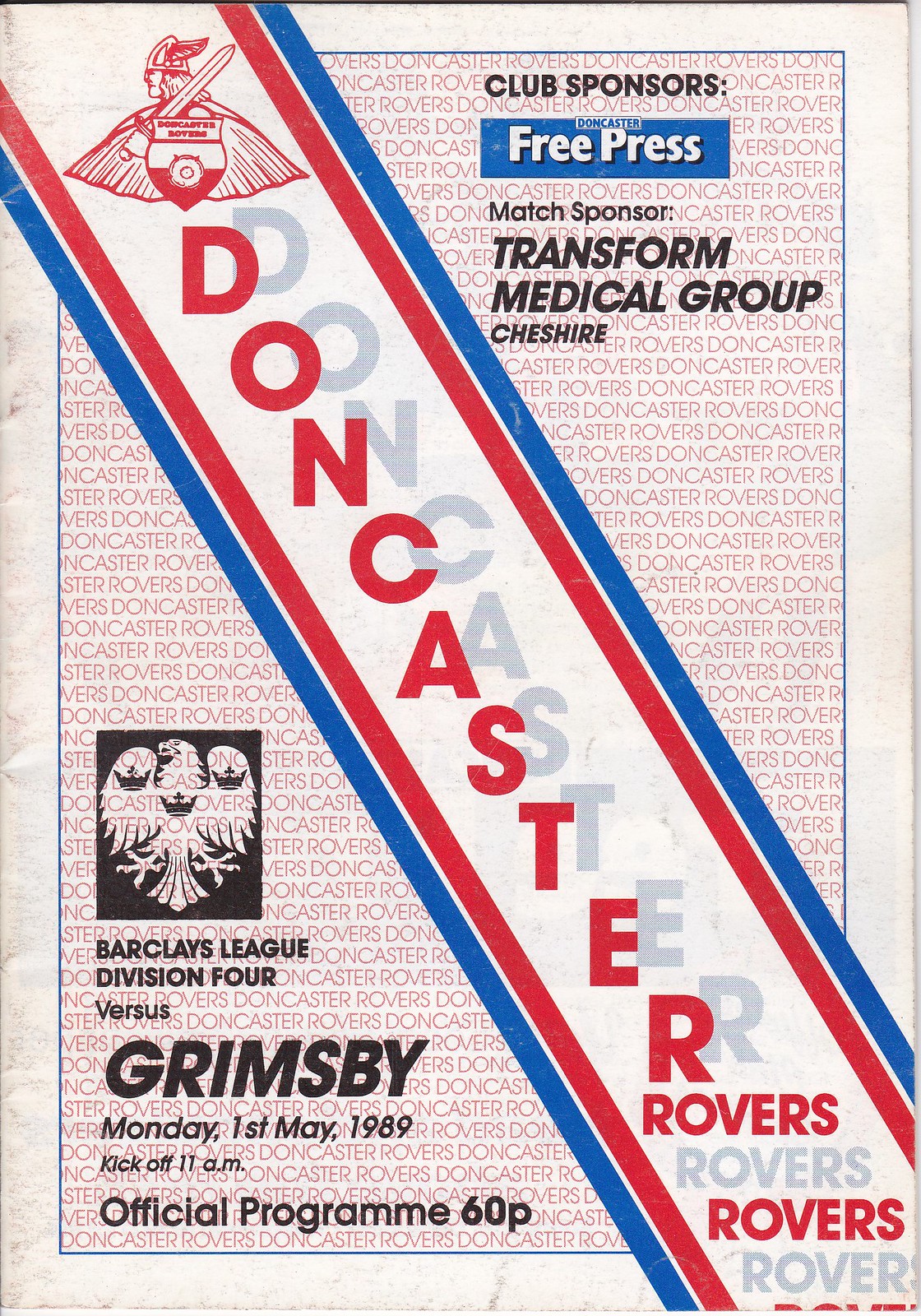The image showcases an old football program from a match between Doncaster Rovers and Grimsby, held on Monday, May 1st, 1989, with a kickoff time of 11 am. The program, priced at 60 pence, features a large diagonal stripe with the word “Doncaster” in shadow lettering prominently across the foreground, written in red. 

Above this stripe, there is the crest of the Doncaster Rovers football club. The crest depicts a warrior, possibly a Viking, wearing a winged helmet, holding a sword, and donning a cape. The shield in the crest features distinct symbols, including letters at the top and a red triangle at the bottom.

Adjacent to the center, the text "Club Sponsors" appears in black. Below this, sponsors listed include Doncaster Free Press, Match Sponsor Transform Medical Group, and Cheshire. A logo of an eagle in the bottom left corner features black text stating "Barclays League Division 4 vs. Grimsby."

Overall, the background is adorned with faint text repeating "Doncaster Rovers," adding depth to the composition. The design elements incorporate red and blue stripes set against a white background, enhancing the vintage aesthetic of the program.